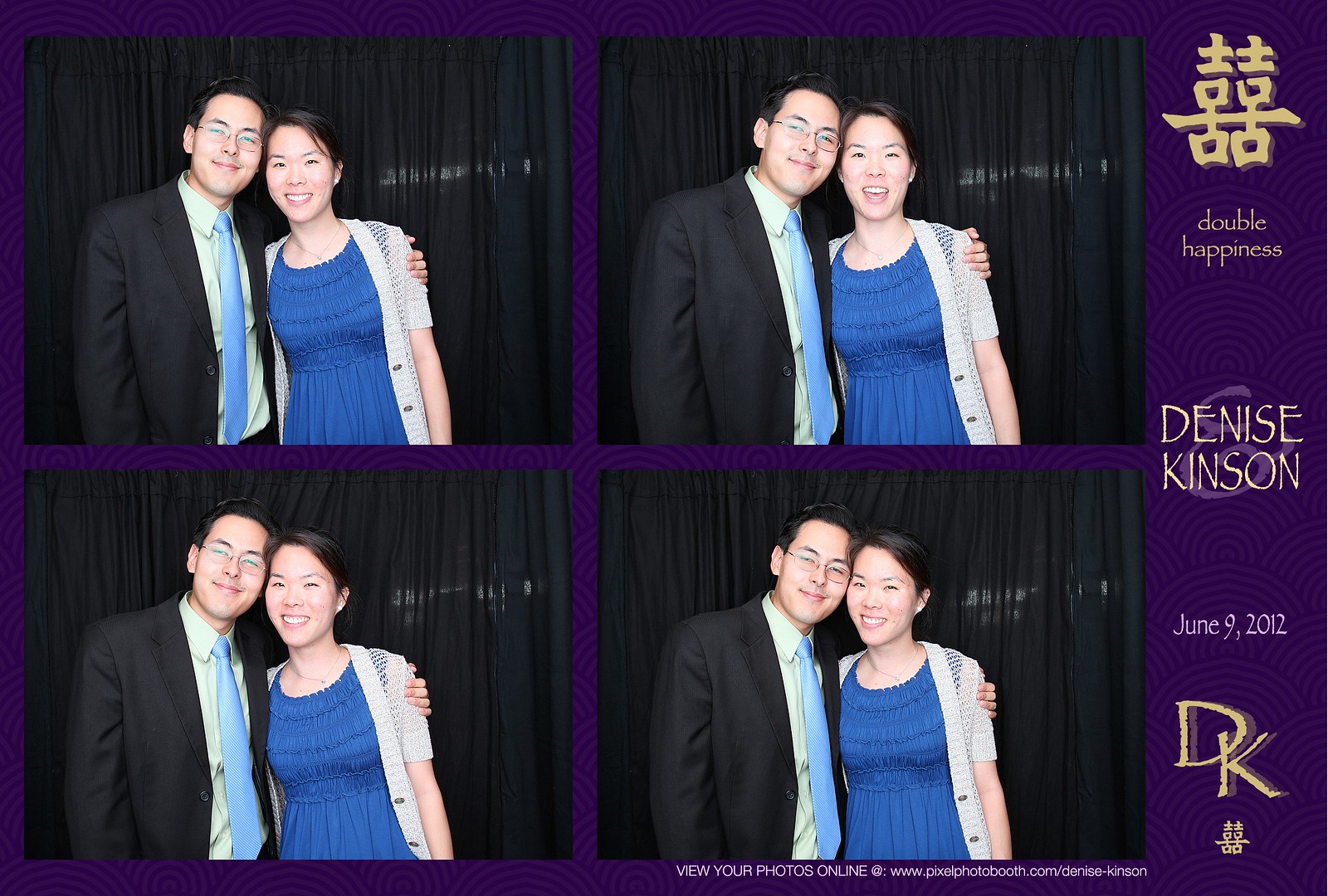A postcard-style photo collage features four snapshots of a happy Asian couple, photographed by Denise Kinson on June 9, 2012. Set against a dark purple background with semi-circular art deco patterns, the images are presented in two rows of two. The man, wearing a black suit, white shirt, and light blue tie, has dark hair and glasses. He lovingly has his left arm resting on the woman’s left bicep. The woman, in a dark blue dress with a white and blue sweater, has dark hair and a radiant smile. Each photo captures the couple with slightly varying expressions, adding a dynamic and intimate feel to the collage. The right side of the image features golden lettering reading "Double Happiness," accompanied by Chinese symbols, the photographer's name Denise Kinson, the date, and the intertwined initials "D.K." At the bottom, there's a link to view the photos online at www.pixelfotobooth.com/denise-kinson.